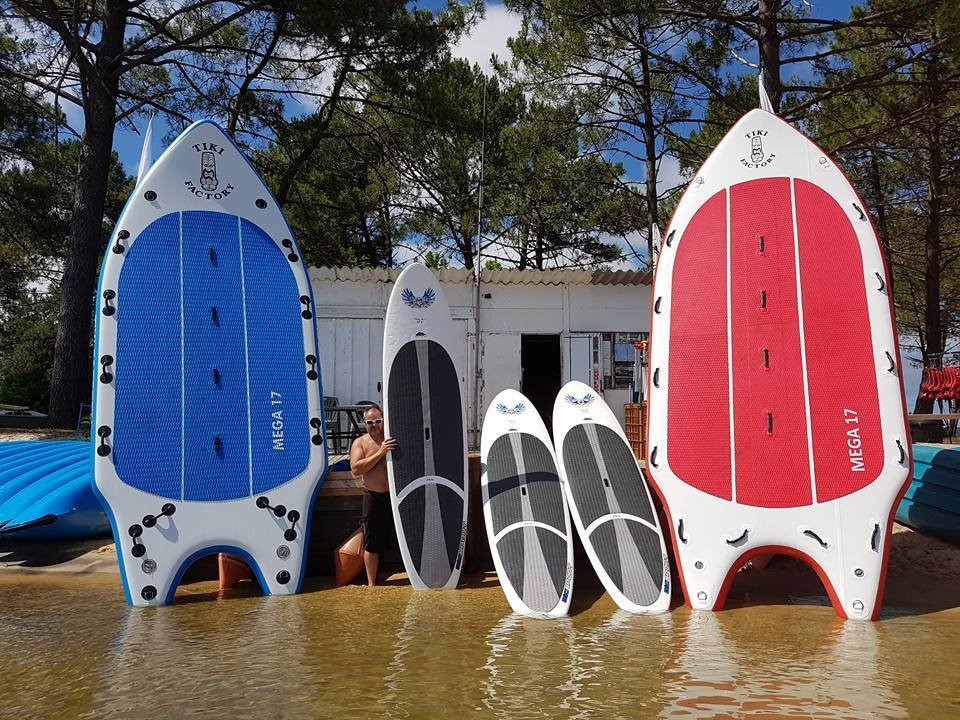The photograph captures a vibrant scene at a water sports business situated beside a lake with brown, rippling water. Dominating the foreground is a shirtless man, wearing black shorts and white sunglasses, proudly holding up a large white paddleboard adorned with a black grip surface. At his feet are two smaller white paddleboards partially submerged in the water and leaning against a dock. To his left stands an impressively tall, 15 to 20 feet, white and blue board emblazoned with the brand name "Tiki Factory." Additionally, several blue kayaks are neatly lined up on the beach to the left.

Behind the man, a rectangular white building with a porch serves as the backdrop, partially hidden by the array of sporting equipment. Adjacent to the building, a rack of life vests is visible, adding to the plethora of gear available for rent or sale. Rolling out to the right are more substantial group-style paddleboards, including another blue one and a red one, both equipped with grips and handles, standing upright with their bases in the water.

Enhancing the picturesque setting, lush pine trees, their green needles shimmering, frame the background against a canvas of blue sky dotted with white clouds. This outdoor image vividly conveys the bustling activity and scenic beauty of this lakeside sports hub.